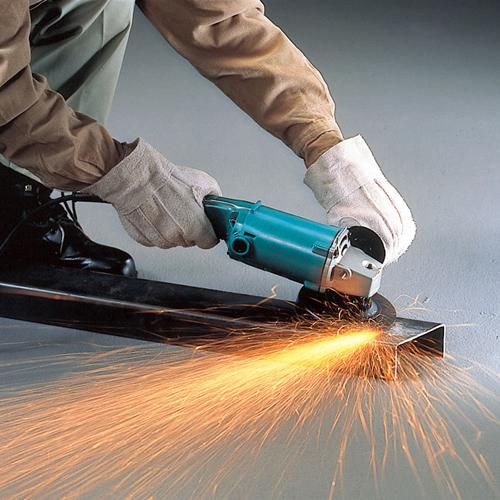In this photograph, a man, partially visible, is engaged in metalwork. He is kneeling in the top left corner, with only his arms and one leg visible. He wears light green pants and a light brown jacket with tan or off-white gloves, and his footwear consists of black shoes. He holds a Tiffany Blue handheld sander against the edge of a large hollow metal beam, which stretches almost across the width of the image. Sparks fly dramatically from the point of contact, creating a vibrant display that occupies a significant portion of the photo's bottom area. The scene is set against a grey background that fades to darker shades in the corners. The man's clothing and gear speak to a heavy-duty work environment, with thick gloves, a sturdy jacket, and robust leather boots, indicative of the protective measures necessary for this high-intensity task.